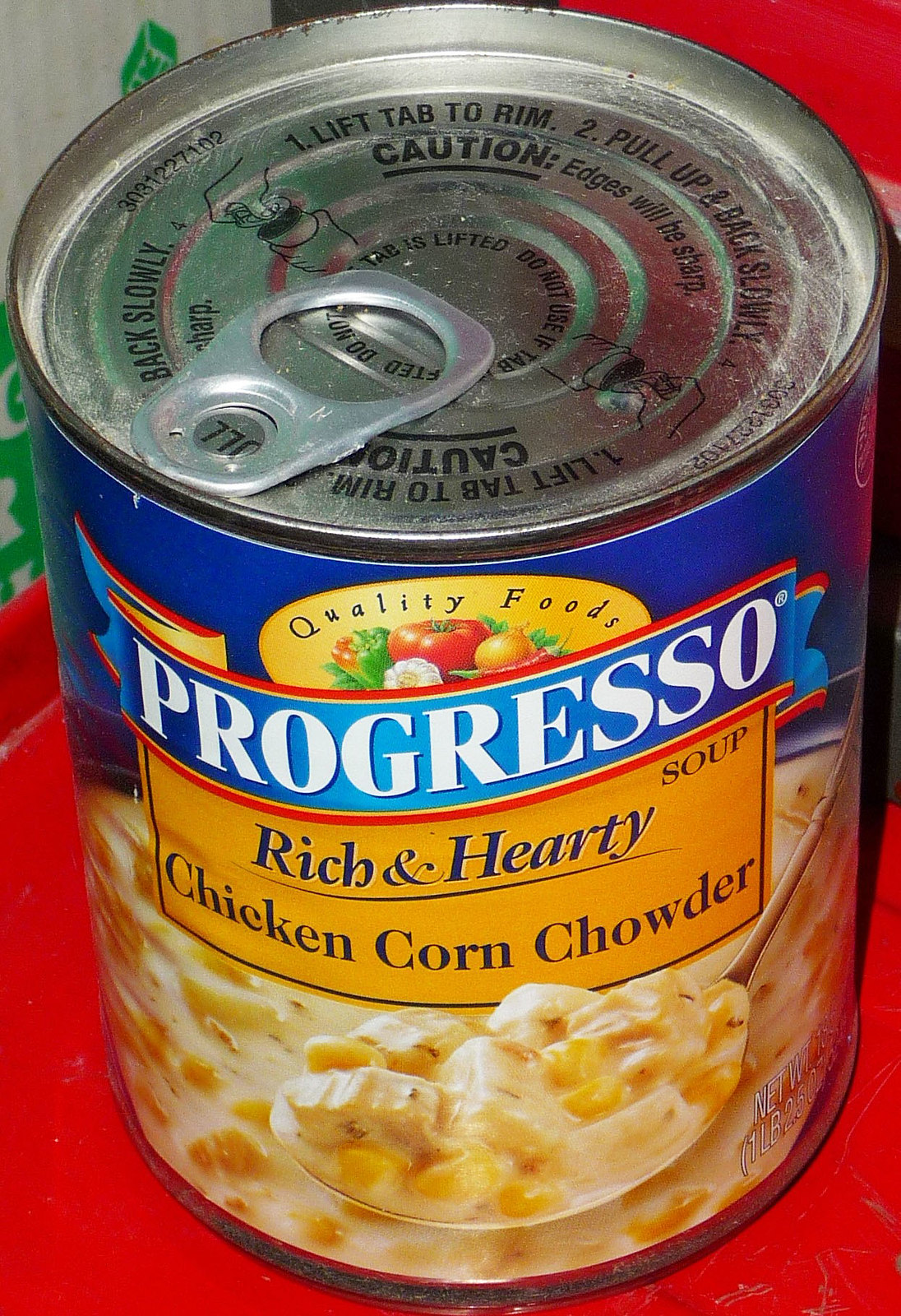A downward-angled photograph showcases a can of Progresso Rich & Hearty Chicken Corn Chowder Soup. The aluminum can features a silver pull tab prominently displayed on its top, accompanied by clear instructions: "1. Lift tab to rim. 2. Pull back slowly. Caution, edges will be sharp." Below the tab, the can's label is visible with vibrant graphics and text. The background of the label is a deep blue, with the "Quality Foods" logo at the top, flanked by images of fresh onions and a ripe tomato. The brand name "Progresso" is boldly presented, followed by the product description "Rich & Hearty Chicken Corn Chowder Soup" in a contrasting font. An appetizing image of the creamy chowder, filled with chunks of chicken and corn, is depicted on the front of the label, enticing viewers. The can is placed on a red table surface, adding a pop of color to the composition. Overall, the photograph provides a comprehensive and appealing view of the soup can.